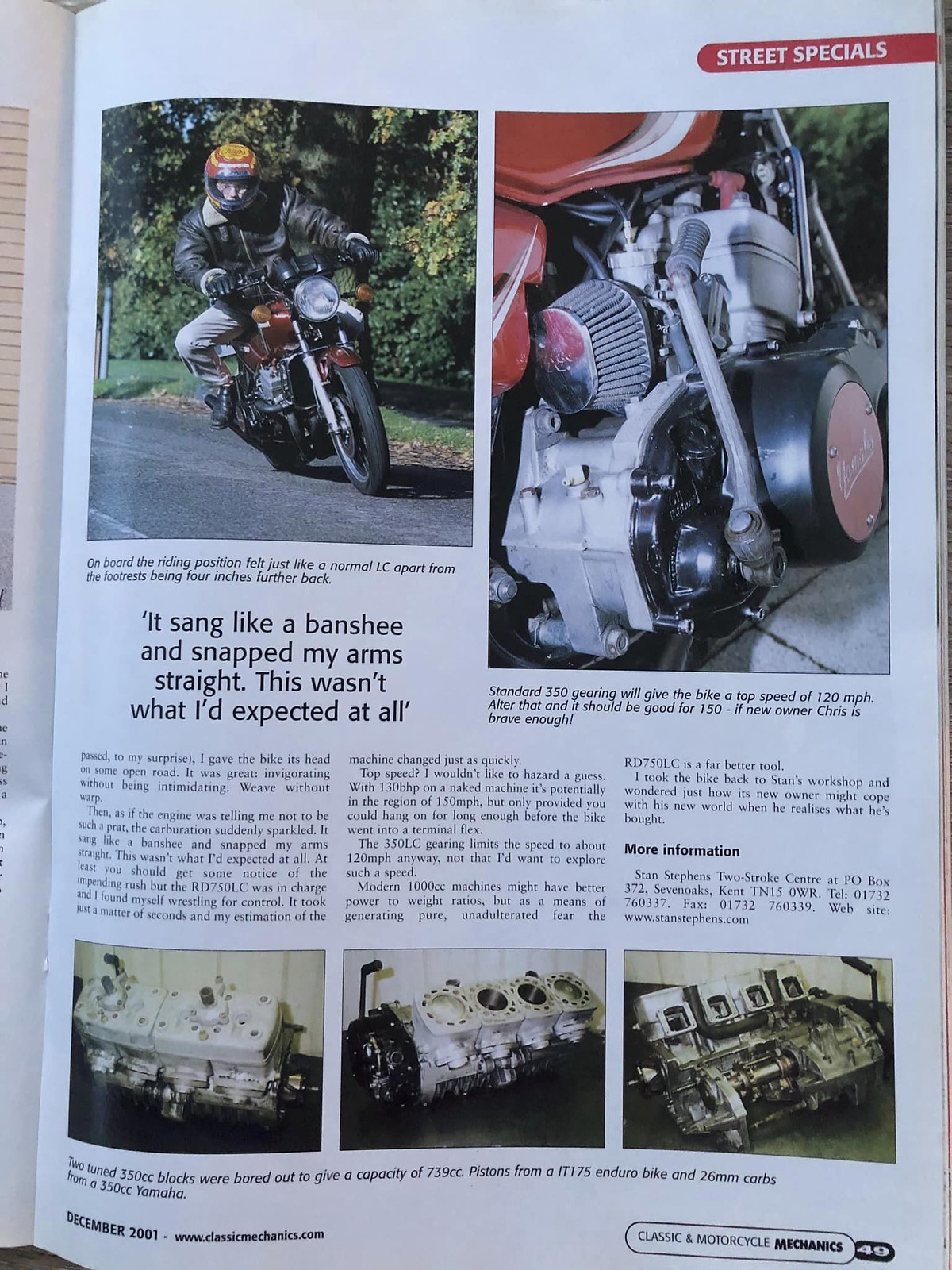This image is a full-color page from the magazine Classic and Motorcycle Mechanics, specifically page 49, featuring an article under the category "Street Specials," prominently displayed in bold red at the top. The layout includes five photographs: 

At the top left, there's a dynamic shot of a man riding a motorcycle, viewed from the front. He is equipped with an orange helmet with a visor, a heavy leather bomber jacket, leather gloves, khaki pants, and boots. Adjacent to this is a detailed close-up of a motorcycle engine, particularly focusing on the air filter or intake. A notable pull quote nearby reads, "It sang like a banshee and snapped my arms straight. This wasn't what I expected at all."

The bottom section of the page features three more photographs, which are part of a detailed look at the engine's internal components. These images illustrate the process of tearing down the engine block. The accompanying caption explains that "Two tuned 350cc blocks were bored out to give a capacity of 739cc, using pistons from an IT175 enduro bike and 26mm carbs from a 350cc Yamaha."

Overall, the article captures both the thrill of riding and the technical intricacies of motorcycle mechanics.